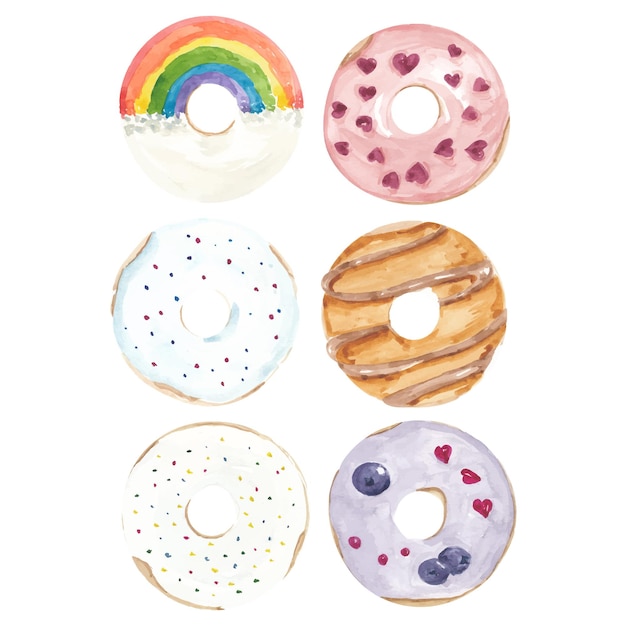This illustration showcases six distinct doughnuts, meticulously organized into 2 columns and 3 rows against a white backdrop. Each doughnut is uniquely decorated, reflecting a vibrant array of colors and patterns. 

Starting from the top left, the first doughnut features a striking design with a rainbow pattern adorning the upper half and a smooth white glaze covering the lower half. Directly below it, the second doughnut is coated with light blue icing and sprinkled with an assortment of colorful dots. The doughnut in the bottom left row follows with a similar design, yet with white icing and a more delicate sprinkle decoration.

On the top right, the fourth doughnut is enveloped in pink frosting and embellished with whimsical heart shapes. Directly beneath it, the fifth doughnut boasts a rich brown color and a wavy cream pattern gracefully spiraling across its surface. The final doughnut on the bottom right is adorned with light purple icing, interspersed with heart shapes and round decorations in pink and blue hues. Additionally, it features three small blueberries strategically placed around its circular shape, adding an extra touch of visual interest. Each doughnut's distinctive topping and arrangement make for an eye-catching and mouth-watering presentation.